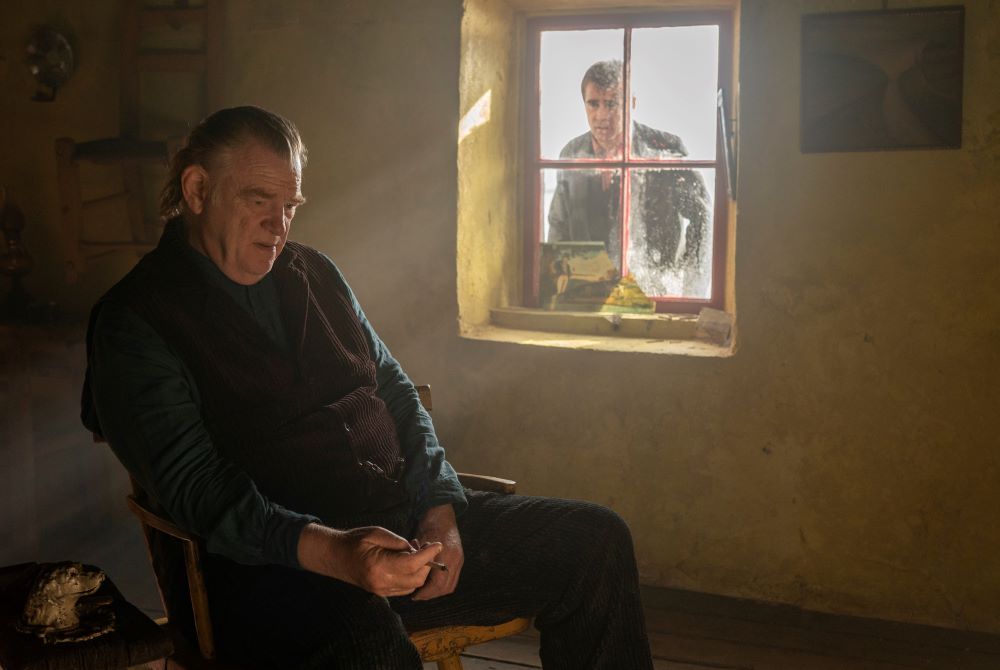In a dimly lit room with yellowish barren walls, an elderly man, likely in his late 70s to mid-80s, sits alone in a brown chair. He dons a brown vest over a teal colored shirt paired with black pants, and his dark gray hair is slicked back. The expression on his face is one of deep sorrow and contemplation as he looks down at an object in his hand, possibly a cigarette. A warm glow from a nearby fireplace casts a subtle light on his face and hands, adding to the melancholic atmosphere of the scene. To the man's left, a window with a distinctive red frame divided into four panes allows light to filter into the room. Outside this window, a young man peers in with a worried and concerned expression, trying to connect with the forlorn figure inside. The background beyond the window fades into a vague grayish-white, adding to the sense of isolation and despair that permeates the image, which seems meticulously crafted, almost like a still from a thoughtful, emotional movie scene.